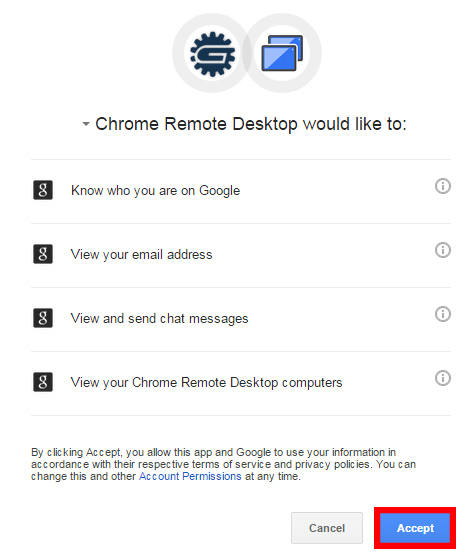The image displays a tablet screen featuring a prompt from Chrome Remote Desktop. The dialog box communicates that the application is requesting permission to access various pieces of information from Google, including the user's identity, email address, chat messages, and Chrome Remote Desktop devices. The message informs the user that by clicking "Accept," they grant the app permission to use this information in accordance with their respective Terms of Service and Privacy Policies. It also notes that account permissions can be modified at any time. Below the message are two buttons for user action: a "Cancel" button contained within a gray rectangle, and an "Accept" button highlighted in a blue box with a red outline. The text on the "Accept" button is written in white font.